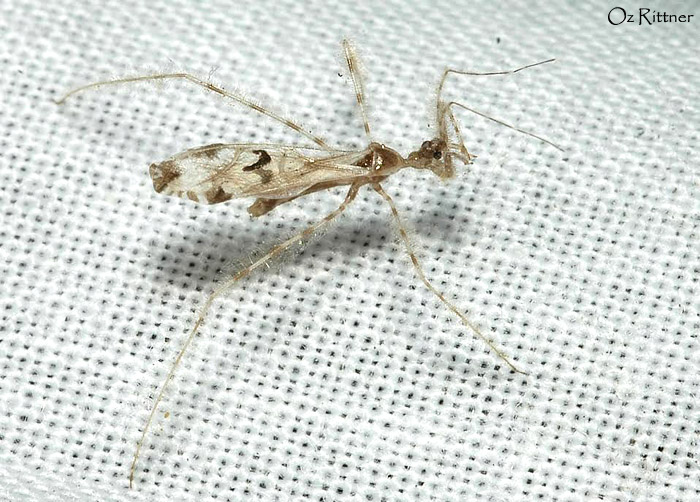The image features a highly zoomed-in perspective of a mosquito, dominating the center of a white mesh grid. The mosquito's body is a mix of whitish and tan hues, highlighted by darker brown symmetrical patterns. Its narrow, elongated body has wings folded across its back, with the wings showcasing extra brown detailing, especially towards the middle and end. The insect's four extremely long legs starkly contrast against the white background, featuring a striking striped pattern of brown and white segments, reminiscent of a candy cane. Additionally, the mosquito’s small brown head flaunts a visible black eye and two long, bent antennae. Written in small font in the top right-hand corner is the name "Oz Rittner."